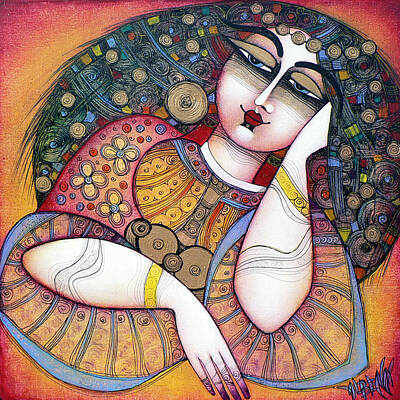This square-shaped painting features a striking gradient background that transitions smoothly from vivid red in the corners to warm orange and bright yellow as it approaches the center. Dominating the center of the canvas is a portrait of a female figure with fair complexion and long, black hair adorned with a myriad of geometric shapes in various colors: beige circles, red triangles and squares, as well as orange and green rectangles.

The woman's head is tilted gently towards the upper right corner, giving a dynamic sense of movement to the composition. Her attire is equally vibrant and intricate, decorated with an array of shapes and patterns mirroring the palette of her hair and background. The shirt includes yellow and blue flowers, red and blue circles, and beige rectangles, creating a harmonious yet lively aesthetic that ties the entire artwork together.